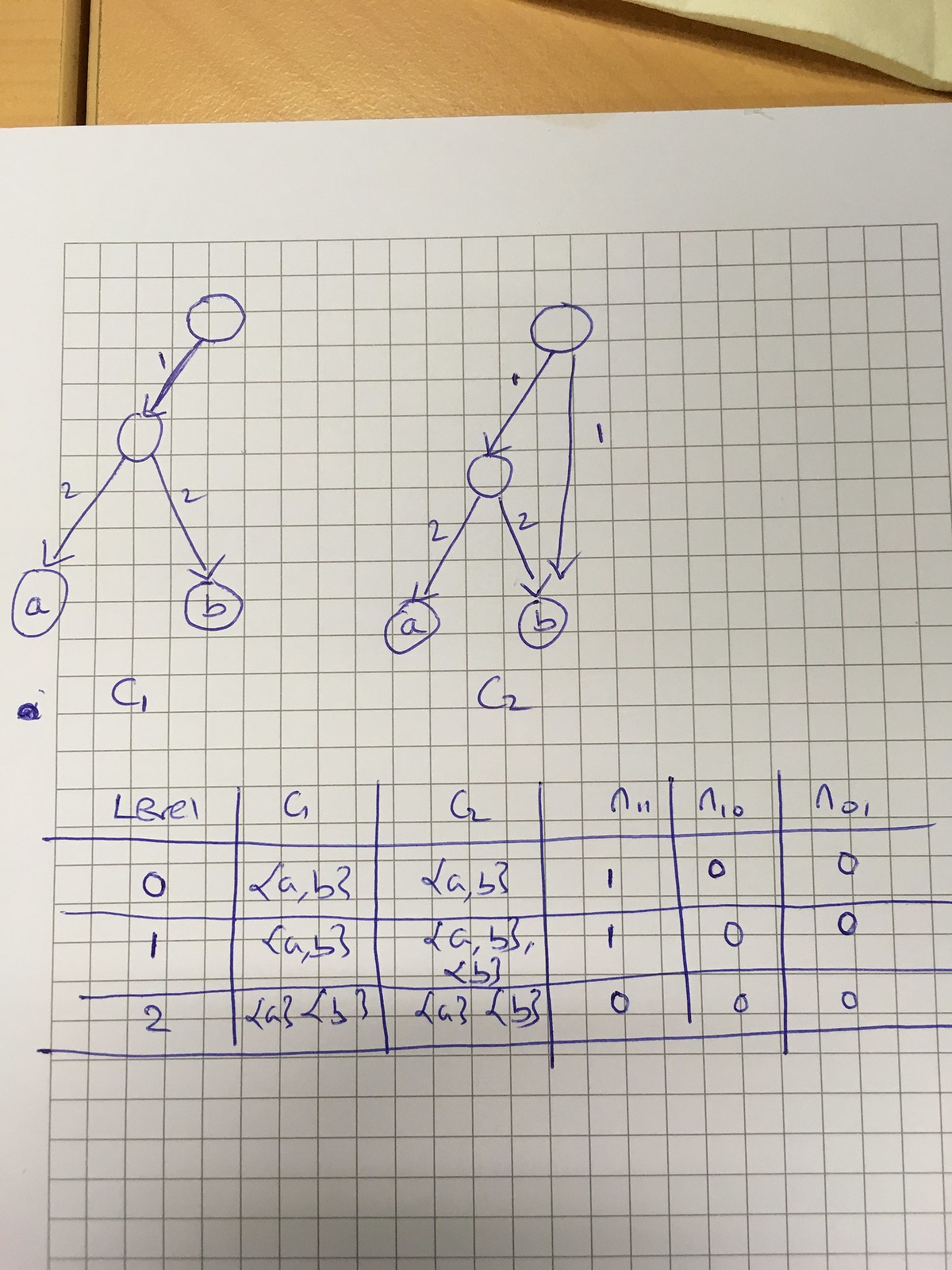This is a detailed diagram sketched on white squared paper, placed against a brown background. The diagrams are meticulously drawn using blue ink. At the upper section of the page, there are figures that resemble stickmen. Each figure consists of a triangle at the bottom, a circle at an angle, and various points connected by arcs. The points are interconnected by curves and are marked with different numbers.

At the bottom of the diagram, two specific points are highlighted and labeled as points A and B, with arrows pointing towards them for emphasis. The two top diagrams are identical except for a subtle difference: the second diagram includes a downward arrow from the upper circle to point B, accompanied by the number one.

Below these figures, there's a chart labeled with levels ranging from 0 to 2, which includes symbols that are not immediately recognizable. These symbols likely hold significant meaning for someone familiar with the concepts being illustrated in the diagram.